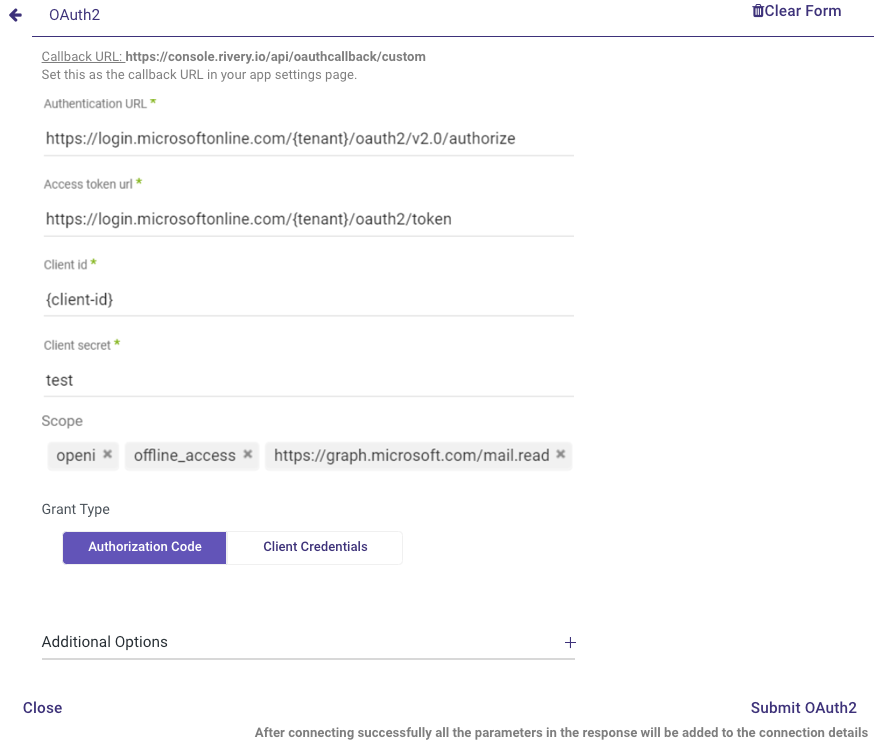The image features a website interface designed for testing OAuth tokens, displayed on a white background. At the top of the interface, there are fields for entering a callback URL and an authentication URL. Below these, the form lists the access token URL, requiring the user to specify a client ID and a client secret to proceed. The headings for each section are in gray, providing clear labels for the input fields, which currently contain placeholder values.

Once the necessary details are filled out, users can generate an authorization code and proceed to log in using these credentials. This process is part of the OAuth protocol, often used to enhance security for applications that do not demand explicit user credentials directly, instead managing them securely behind the scenes.

Additional options can be configured at the bottom of the form, although they are not mandatory. There are several buttons for user interaction: a "Close" button located in the bottom left-hand corner of the screen, a "Clear Form" button at the top right-hand corner, and a submission button at the bottom right-hand corner to finalize and submit the OAuth token.